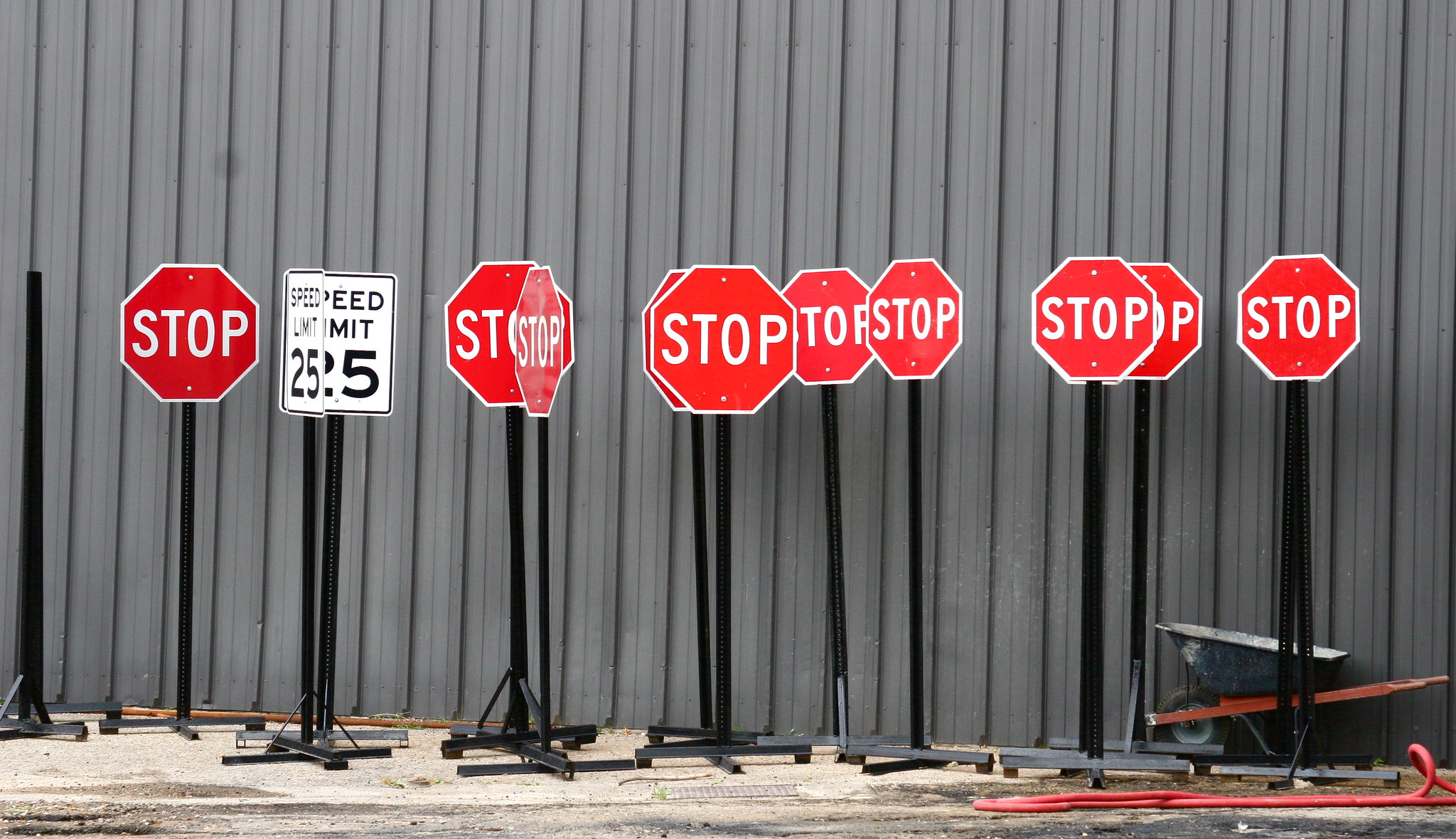The photograph captures an outdoor scene taken during the daytime, showcasing an unusual assembly of road signs. At the forefront, there are ten standard red octagonal stop signs, each displaying the word "STOP" in white. Among these stop signs are also two speed limit signs indicating a limit of 25 mph. All the signs are mounted on tall, narrow black metal posts, which are supported by crossed bases to keep them upright. Behind the cluster of signs is a gray metal or tin wall with a textured surface that features recessed and raised portions. The ground beneath the signs is a concrete sidewalk. In the background, a wheelbarrow and a red pipe can be seen, adding to the industrial feel of the setting. One of the posts standing alone without any sign attached further accentuates the peculiar arrangement.